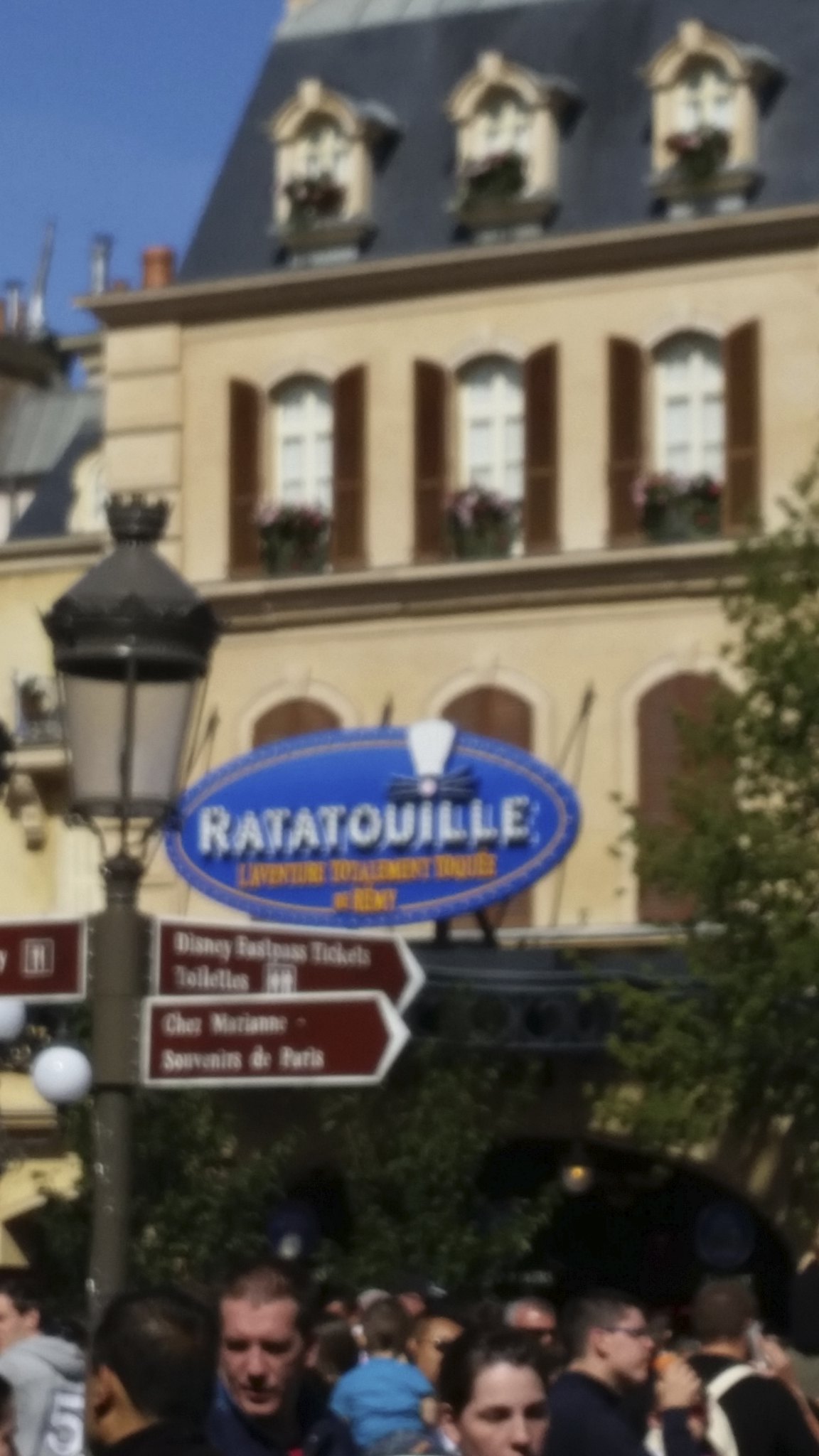The photograph appears to be a very zoomed-in, out-of-focus snapshot taken in portrait mode at one of the Disney theme parks, likely Disneyland Paris. The central feature is a blue oval sign prominently displaying the text "Chez Marie, Souvenirs de Paris," possibly an advertisement for a Ratatouille-themed attraction or restaurant. The scene also includes a black lamppost with multiple directional signs—some clearly pointing to "tickets," "toilets," and one partially-readable sign suggesting "Disney Express." The backdrop reveals a charming French-style courtyard bustling with visitors, featuring a white chateau-like building adorned with large brown window shutters and cut-out roof windows, all under a bright blue sky peppered with trees.